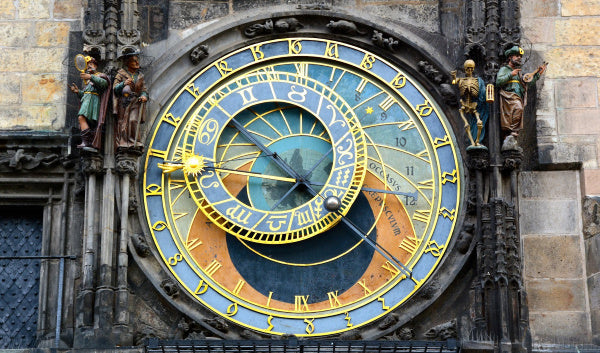This photograph showcases a large, intricately designed clock mounted on the exterior wall of a building constructed with gray and brown bricks. The clock, notable for its circular shape and predominantly blue face, features multiple time-telling methods. Golden yellow characters stand out vividly against the blue background, including a 24-hour format featuring numbers from 1 to 23. Additionally, Roman numerals and Arabic symbols also represent the hours within the same clock face. The face of the clock is bordered by smaller, vibrant elements in orange, dark blue, and yellow. A smaller wheel, or sub-dial, is nested within the main clock, adding another layer of detail. Flanking the clock are small statues, or figurines of men, enhancing the elaborate design.